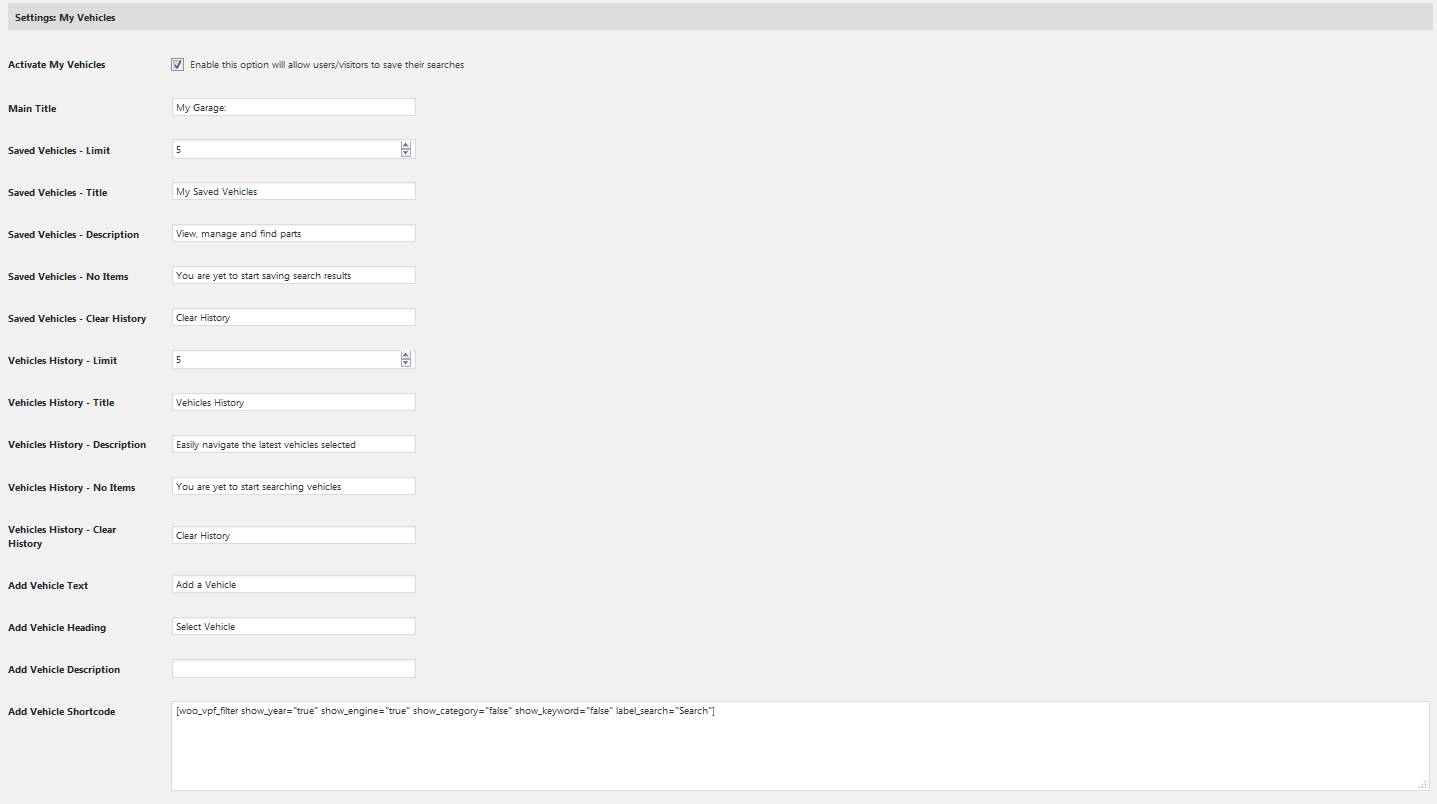This image displays a grayish-colored screen featuring a detailed settings interface labeled "Settings" in the top left corner. Below this header, the left side of the screen lists multiple configuration options sequentially from top to bottom.

1. **Activate My Vehicles**: Accompanied by a checkbox, enabling this option allows users or visitors to save their searches.
2. **Main Title**: Define the primary heading.
3. **Saved Vehicles Limit**: Set the maximum number of vehicles that can be saved.
4. **Saved Vehicles Title**: Title for the saved vehicles section.
5. **Saved Vehicles Description**: Description for the saved vehicles section.
6. **Saved Vehicles No Items**: Message displayed when no vehicles are saved.
7. **Saved Vehicles Clear History**: Option to clear the saved vehicles history.

The list continues with similar settings for vehicle history:

8. **Vehicle History Limit**: Limit the number of historical vehicle entries.
9. **Vehicle History Title**: Title for the vehicle history section.
10. **Vehicle History Description**: Description for the vehicle history section.
11. **Vehicle History No Items**: Message displayed when there is no vehicle history.
12. **Vehicle History Clear History**: Option to clear vehicle history.

Settings for adding new vehicle entries include:

13. **Add Vehicle Text**: Text for adding a new vehicle.
14. **Add Vehicle Heading**: Heading for the add vehicle section.
15. **Add Vehicle Description**: Description for the add vehicle section.
16. **Add Vehicle Shortcode**: A large white box to the right where a shortcode can be entered. This box contains black text and can be expanded via an option at the bottom right corner.